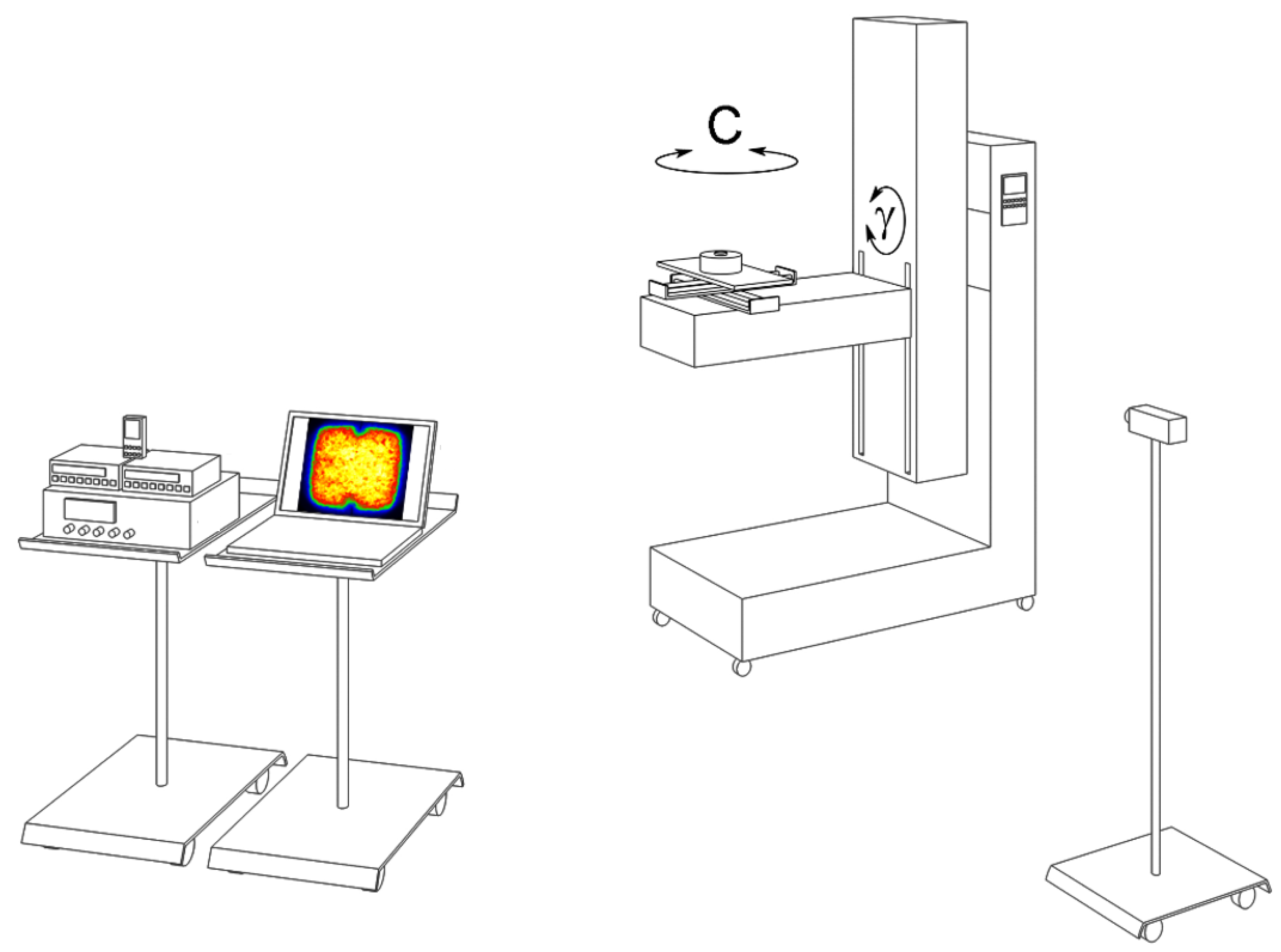This detailed line drawing, predominantly in black and white, showcases various pieces of equipment that appear to be medical devices. The scene features a total of four key items, illustrated with an emphasis on precise outlines and minimal coloring. Positioned in the bottom-left corner is an open laptop resting on one of two portable podiums. This laptop screen stands out with a distinct depiction of a colorful image, resembling a cross-section of a brain with a dark exterior, vibrant blue outline, and a mix of bright yellow and reddish-orange hues. Adjacent to the laptop podium is a table hosting a machine that bears a resemblance to an old-fashioned stereo system, possibly with a cell phone placed on top.

Moving towards the center and right side of the image, there is another machine characterized by an L-shaped base and an arm that supports a vertically adjustable shelf, featuring a rotating component marked with a 'C' and surrounded by two circling arrows. This component might be associated with x-ray or MRI functionality, or even a mammography device. Additionally, in the bottom-right corner of the drawing, a platform with a pole surmounts a small element that could potentially be part of a camera setup, akin to a video recording device. The detailed yet simplistic nature of the drawing highlights the functional aspects of these medical apparatuses, suggesting a clinical environment.